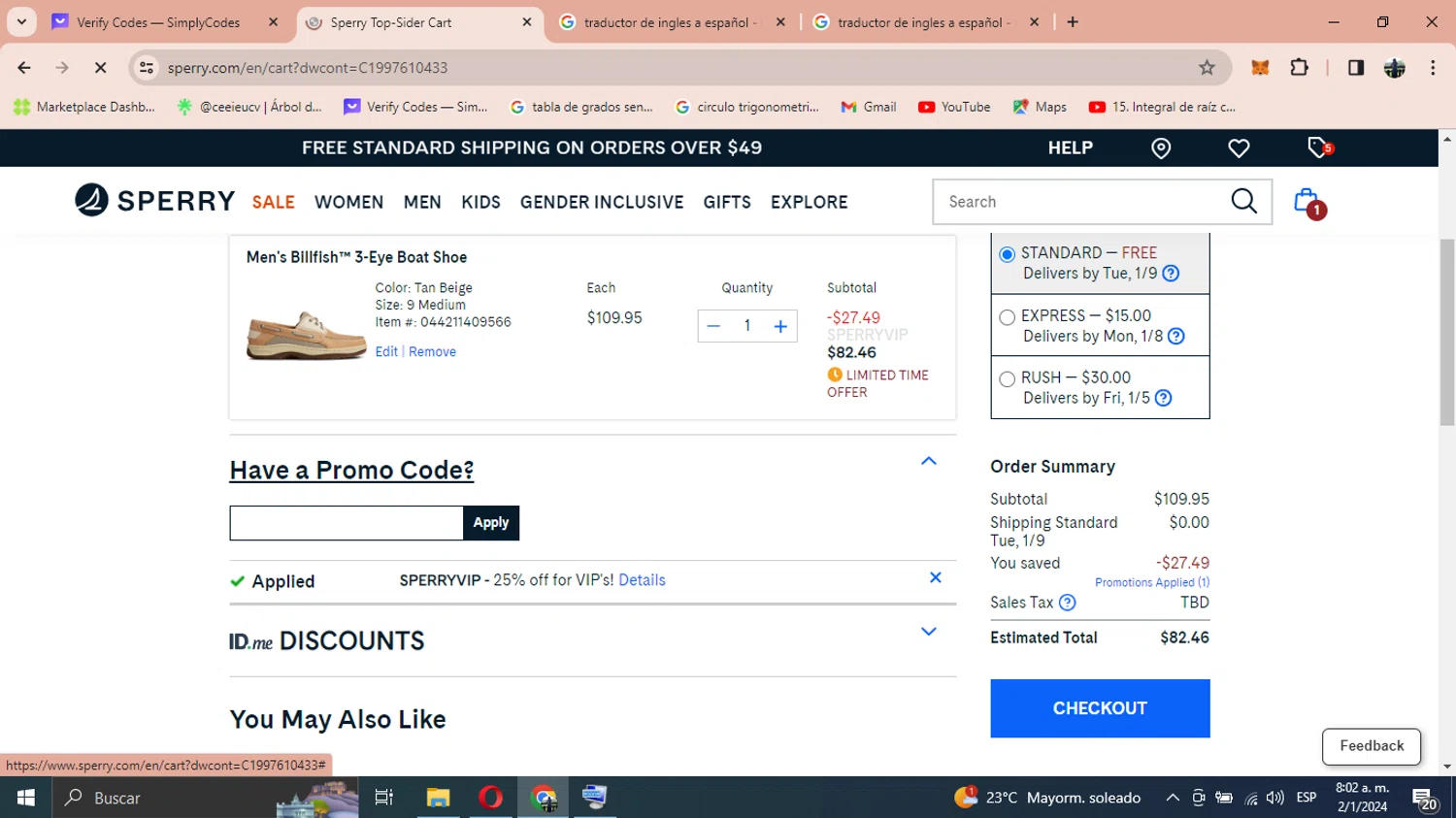The image depicts a detailed screenshot of a Windows computer screen. The layout is unmistakably Windows, as indicated by the Windows logo situated in the bottom left corner. Adjacent to the logo is the search bar with a magnifying glass icon followed by the text "Best Bar." Next to these, is an icon depicting the world and monuments which likely represents a web browser home or a similar feature.

Continuing to the right, there is a sequence of icons including a network connection symbol, a folder icon, a red 'O' (probably for Opera browser), a Google Chrome icon, an application symbol showing a computer screen, and a weather symbol indicating 23°C. To the right of these, the text "Mallarm Solado" is displayed.

On the rightmost part of the taskbar, there are additional system icons: network connection, desktop display shortcut, Wi-Fi status, speaker control, ESP (possibly a language setting), the current time (8:02 a.m.), and the date (February 1st, 2024). Notably, there's a notification icon showing 20 pending alerts. The screenshot also includes a vertical scroll bar on the right side.

At the top of the screen, a drop-down arrow is visible along with four open browser tabs. The tabs are labeled as follows:
1. "Wi-Fi code, Simply Codes"
2. "Ferry, Top Slider Cart, X" (the active tab)
3. "Traductor de Inglés a Español" (with an X sign)
4. Another identical tab "Traductor de Inglés a Español" (with an X sign).

The content of the screen is centered on the Sperry website, specifically at the checkout page for a men's Billfish 3-Eye Boat Shoe in the color beige, size 9 (medium). The item number is 00044211409566, priced at $109.95 with a quantity of 1. The subtotal is shown as $27.49 after the Sperry VIP discount, bringing the total to $82.46. Standard shipping is selected with an expected delivery by Tuesday, January 9th. The promo code applied, "Sperry VIP," granted a 25% discount for VIP members.